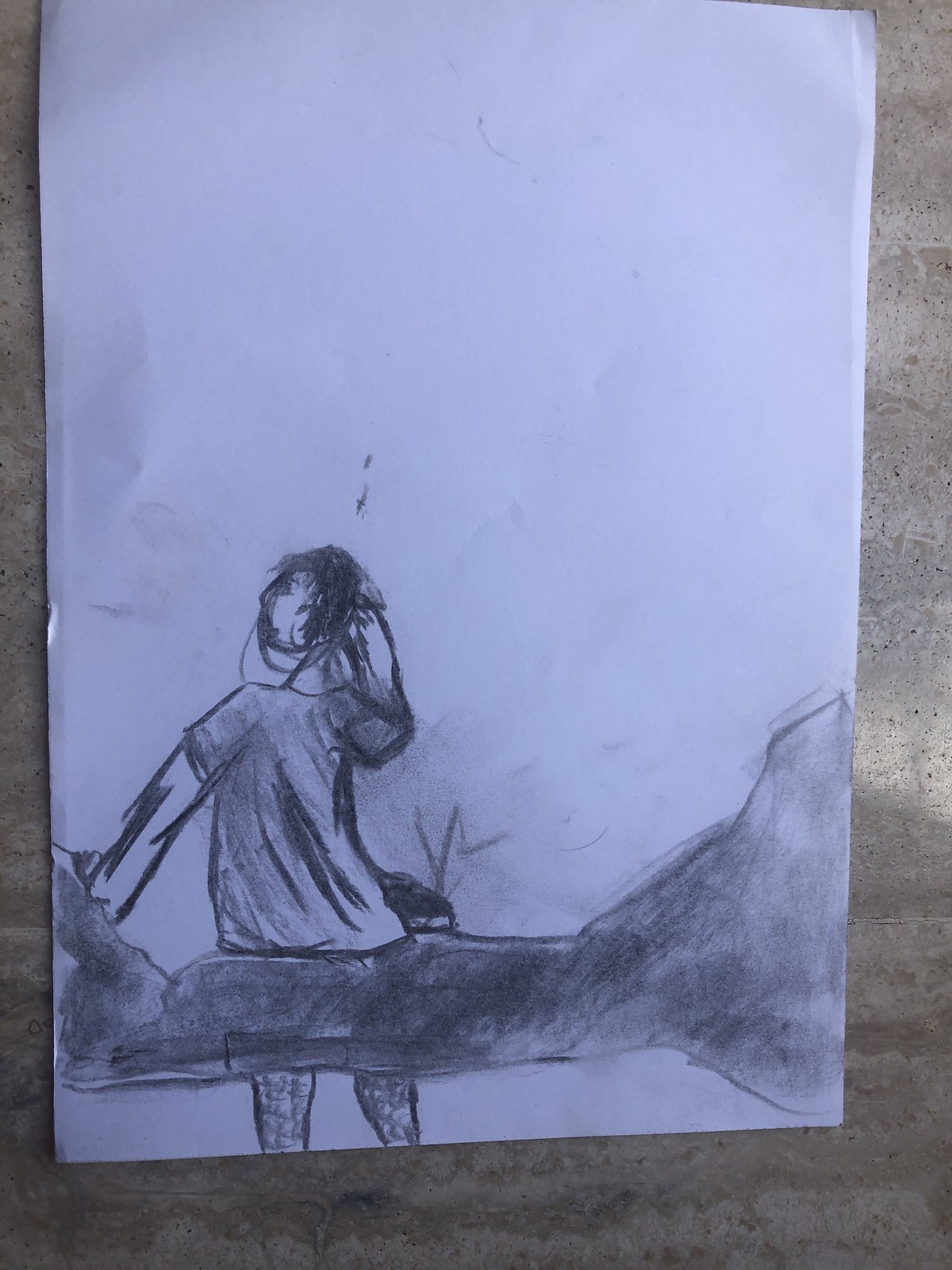The image showcases a detailed pencil drawing on a piece of white paper, which is placed on a brown and beige, marbleized stone or granite surface. At the bottom half of the paper, the drawing depicts a person sitting on what appears to be either a bench or a log. The log is flat in the middle and has raised portions on both the left and right sides, with the right portion being larger. The person, drawn from the back, is facing towards the left. They are wearing a t-shirt shaded in various tones of gray, also done with pencil. From beneath the log, part of the person’s legs are visible, seemingly adorned with socks. The individual's left arm rests on the log while the right arm is raised towards their head. The hair is sketched in detail, and their face, turned to the left, shows a nose, one eye, and part of their mouth.